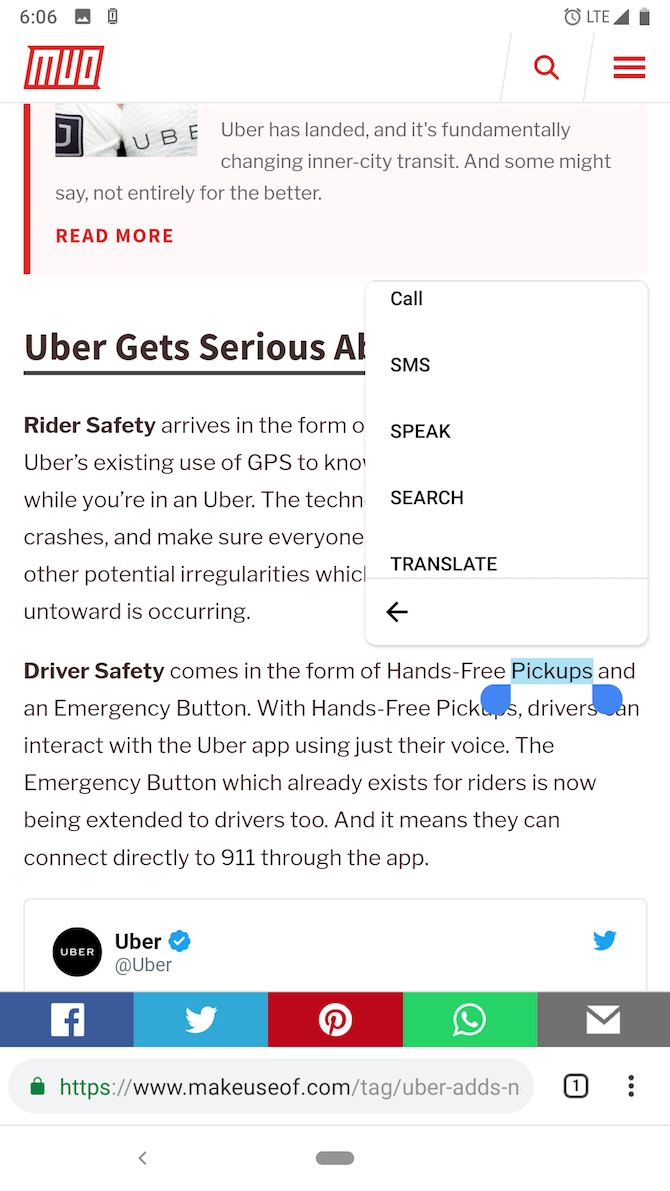The image is a screenshot from a mobile phone. The background at the very top is white with some grey text displaying information about the phone. In the upper left corner, it shows the time as "6:06". Next to the time, there is an icon of a picture, a battery icon, an alarm clock icon, and the text "LTE". Below these icons, a webpage is open. 

At the very bottom of the screen, there is a navigation bar displaying the webpage address: "https://www.makeuseof.com". Above this bar is an article with the headline "Uber has landed and it's fundamentally changing inner city transit. And some might say not entirely for the better. Read more." Directly below the headline and continuing within the article, there is a small pop-up menu in the form of a white vertical rectangle with black text. This menu contains the options: "call, SMS, speak, search, translate," listed vertically. Additionally, there is a small arrow pointing left. Further down, the article continues with the title "Uber gets serious about safety."